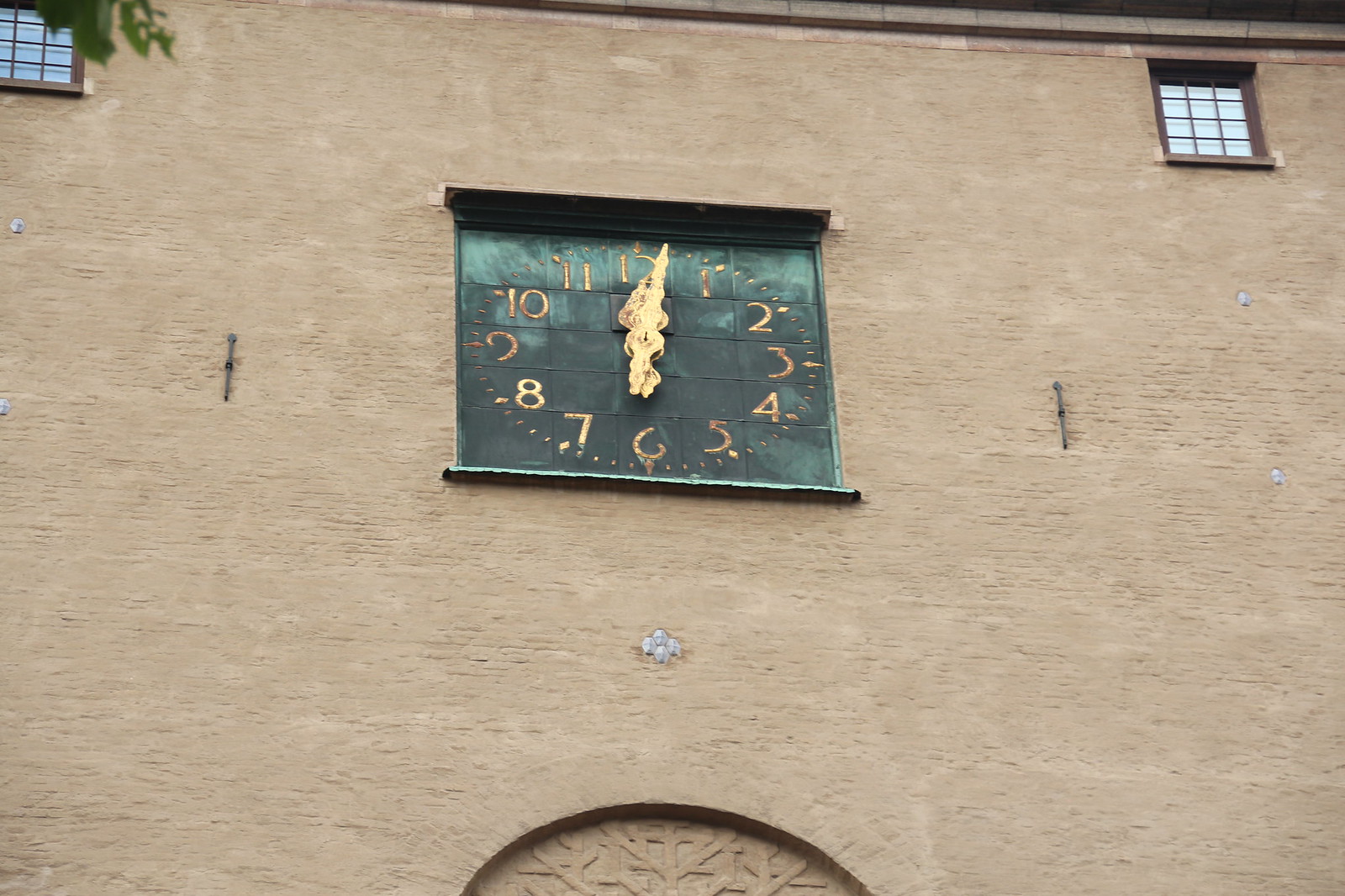The image captures an upward view of an exterior wall of a light brown brick building, emphasizing intricate architectural details. At the bottom of the image, there's a semi-circular archway adorned with a twig-like design pattern, partially visible and suggesting it might be an entrance. Above the archway, four hexagonal metal light fixtures are aligned closely together. Dominating the middle section of the wall is a square, rusted clock with a green face, featuring distressed gold numbers and hands, hinting at once having a more pristine appearance. The clock frame is bordered at the top and bottom. The building's upper section showcases two brown framed windows, one on each corner, with brown bars or squares within them. The background is visible in parts, showing a green hue behind the clock, with the numbers and clock hands tarnishing to brown due to rust. The top of the building is lined with a lighter gray border, and a small portion of a tree branches into the view from the top left corner, adding a touch of nature to the urban structure.